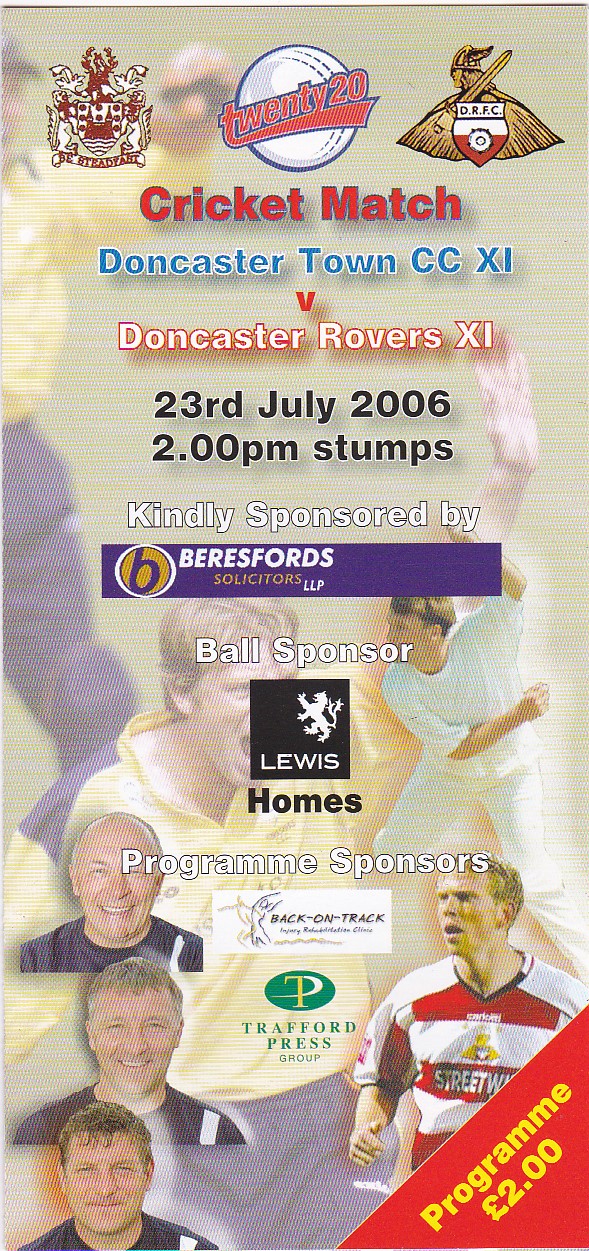The front page of this program for a cricket match features a narrow, pamphlet-style layout with a somewhat faded background image of soccer players, including one prominent player and a coach. At the top, there are three logos: the central one is a soccer ball with "2020" in red letters, flanked by a team logo depicting a Viking with a sword and a crest with lions. Below, the program details the cricket match between Doncaster Town CC XL and Doncaster Rovers XL, scheduled for 23rd July 2006 at 2 PM at The Stumps. Sponsors are prominently mentioned: Beresford Solicitors in a purple banner, Lewis Holmes as the ball sponsor, and Back on Track along with Trafford Press Group as program sponsors. The bottom corner indicates that the program costs two British pounds. The design also features a collage of player and participant faces, adding a personal touch to the informative layout.